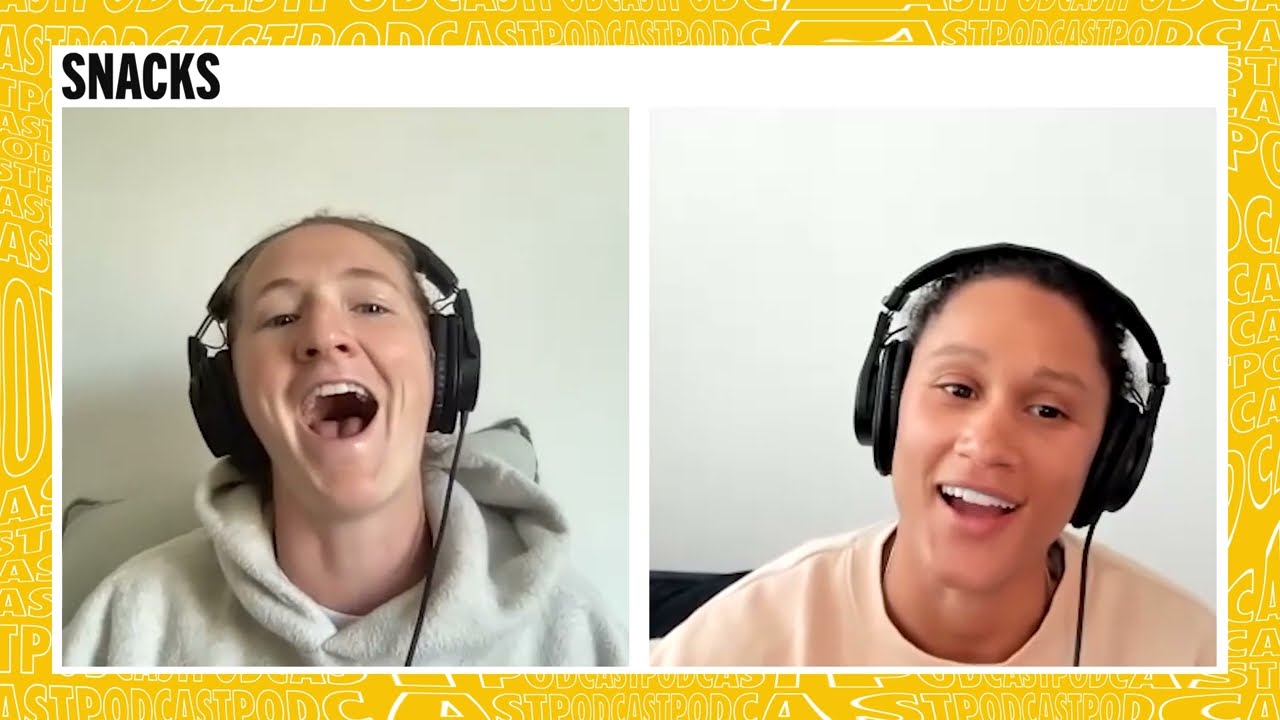The image is split into two parts and appears to be a promotional screenshot, possibly from a YouTube video or podcast. It features two women, each in their own segment with a shared yellow border around the entire image. At the top left, the word "SNACKS" is written in bold black, capital letters, and beneath it, repeating white bubble letters spell out "PODCAST" against a gold background.

On the left side, the woman is wearing a cozy white hoodie and black headphones with a wire coming out of the right side. She has short blonde hair, light brown eyebrows, and a pale complexion. Her head is thrown back, mouth wide open, showing her teeth and appearing to laugh heartily. The background behind her is a very light blue or white.

On the right side, the other woman is also wearing black headphones and a light beige or off-pink sweater. She has darker hair and eyes and a slightly darker complexion compared to the woman on the left. She is smiling with her mouth partially open, showing her white teeth but not as wide as the woman on the left. Her background is similar in color, and a black couch is visible to her lower right.

Both women are seated in front of a white or very light blue wall and appear happy, suggesting they are enjoying a moment together, possibly during a podcast recording.